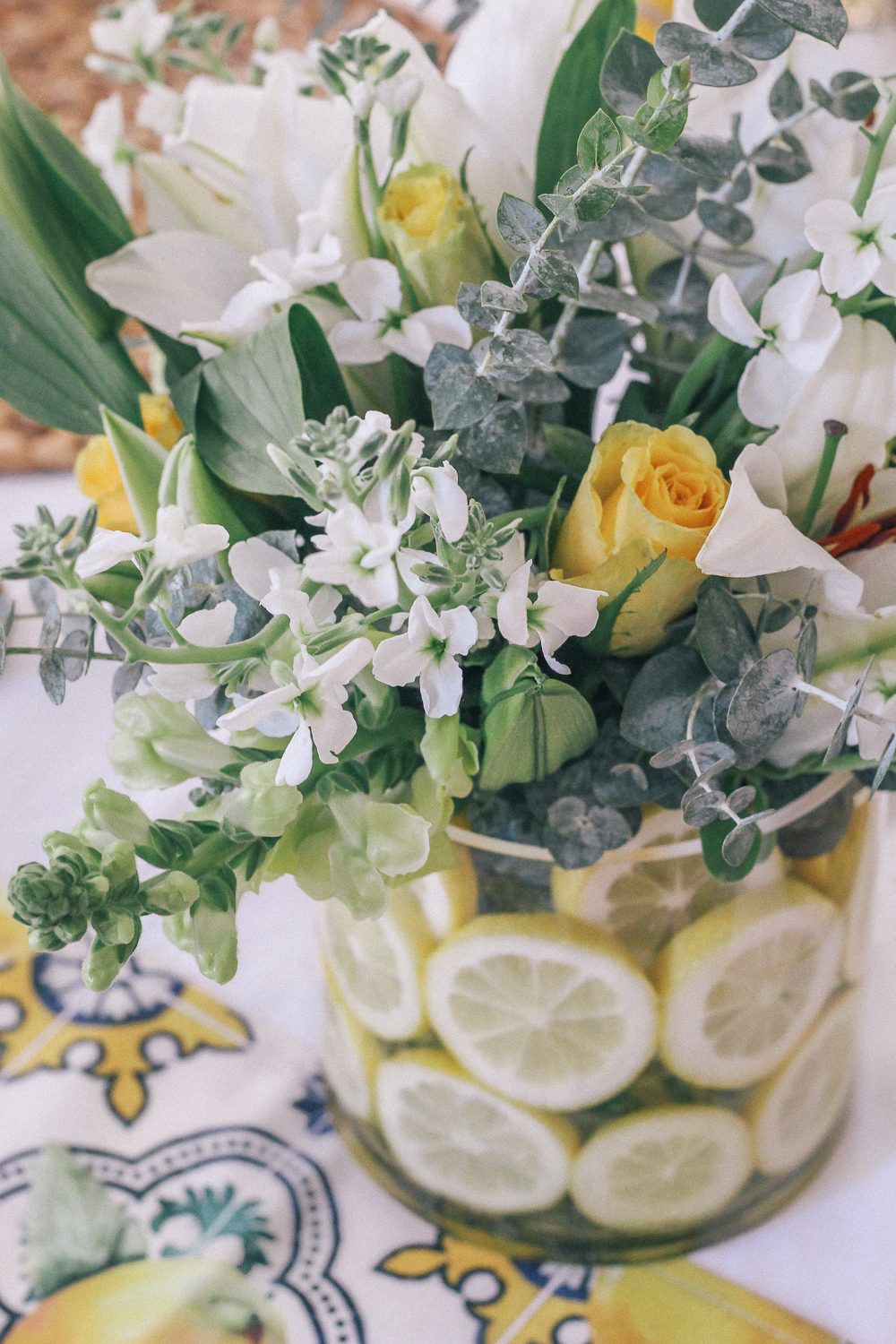The image is a close-up photograph of a tall, rectangular arrangement that serves as a table centerpiece. The centerpiece consists of a transparent glass vase filled with sliced lemons, arranged vertically and lining the inner walls of the vase, creating a circular, wheel-like pattern. Inside the vase, intermingled with the lemons, is a vibrant bouquet featuring yellow roses, white flowers, and an assortment of green leaves and stems. The vase rests on a white tablecloth adorned with intricate yellow and blue designs, which include flowery motifs and half-sailor wheel patterns, adding to the overall aesthetic of the composition.